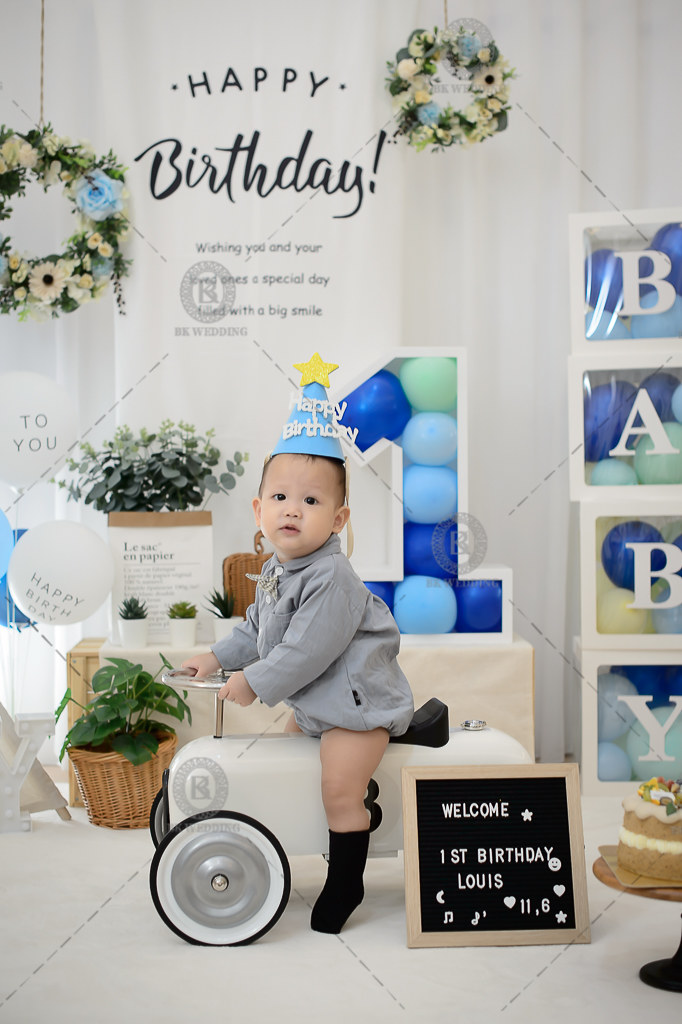This vibrant image captures the joyous celebration of a baby named Louis at his first birthday party. Louis is beaming at the camera while riding a small, white car with a steering wheel. He is dressed in a cozy gray outfit, topped with a blue hat emblazoned with "Happy Birthday" and a yellow star. Surrounding him are festive elements that amplify the celebratory atmosphere: 

- A "Welcome First Birthday, Louis" sign prominently displayed, adding a personalized touch.
- "HAPPY BIRTHDAY" prominently written in an eye-catching design, with "HAPPY" in a bold arc and "birthday!" in elegant cursive, complete with an exclamation point.
- Two decorative wreaths hanging from the ceiling, adorned with green leaves, yellow, and blue flowers, enhancing the festive decor.
- Brightly colored balloons in shades of blue, green, and light blue contribute to the cheery ambiance.
- Stacked blocks spelling out "BABY" beside Louis, emphasizing the adorableness of the occasion.

This detailed and heartwarming snapshot captures the essence of a memorable and joyful first birthday celebration, full of unique and playful elements.